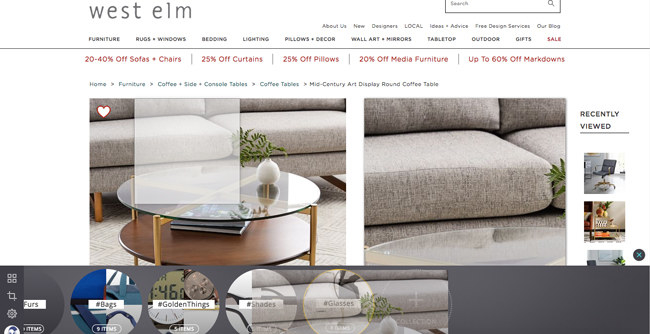Screenshot from the West Elm Website:

The screenshot captures the homepage of the West Elm website, a retailer specializing in home furnishings. At the top, the simple, lowercase West Elm logo is visible. In the upper right corner, there is a search field. Directly below the search bar are navigational links including "About Us," "New Designers," "Local," "Ideas/Advice," and "Free Design Services on our Blog."

The main menu, positioned just beneath these links, lists categories such as Furniture, Rugs, Windows, Bedding, Lighting, Pillows, Decor, Wall Art, Mirrors, Tabletop, Outdoor, Gifts, and Sale (highlighted in red). Below this menu, a thin gray line separates further promotional areas with vertical gray bars between them. These promotions include "20-40% off sofas and chairs," "25% off curtains," "25% off pillows," "20% off media furniture," and "up to 60% off markdowns."

The page appears to be mid-selection in the "Home Furniture" section, specifically focused on a mid-century modern art display and coffee table selection. It features two main photos: a close-up image on the right showing the glass surface of the table, and a larger image on the left depicting the table in front of a gray sofa.

To the right of these images are thumbnails for recently viewed items. At the bottom of the screenshot are four circled options labeled bags, golden things, shades, and glasses, accompanied by some graphic elements and cropping tools to the left. These additional elements suggest that this screenshot might depict someone actively working on the website, as it includes design and editing tools not typically visible to general users.